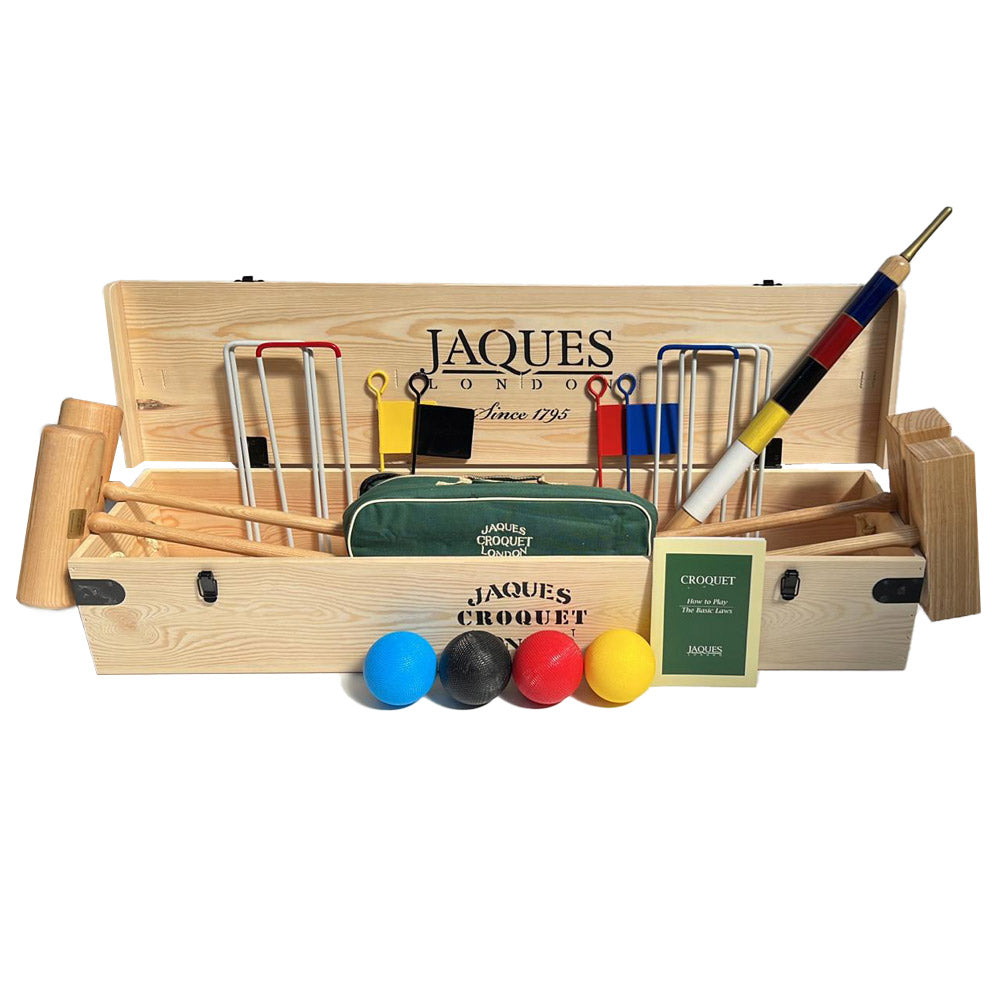This is a detailed photograph of a croquet set displayed on a white background. The main feature is a wooden box labeled "Jackus London since 1795, Jack's Croquet." The box is of a bright wood color, matching the two types of croquet mallets it contains: rounded ones on the left and square-shaped ones on the right, all made of the same bright wood. 

In front of the box, there are four croquet balls arranged from left to right in blue, black, red, and yellow colors. Accompanying the set, there are small wooden flags and arches to be inserted into the ground, some pure white and others tipped with red or blue. Also included is a small army green booklet with a yellow frame titled "Croquet: How to Play," featuring "Jackus" at the bottom. Additionally, there is a zippered case presumably to store the balls and protect them from bouncing around and damaging other parts inside the box. This detailed croquet set appears ready for a classic game, thoughtfully designed with both functionality and aesthetic appeal.